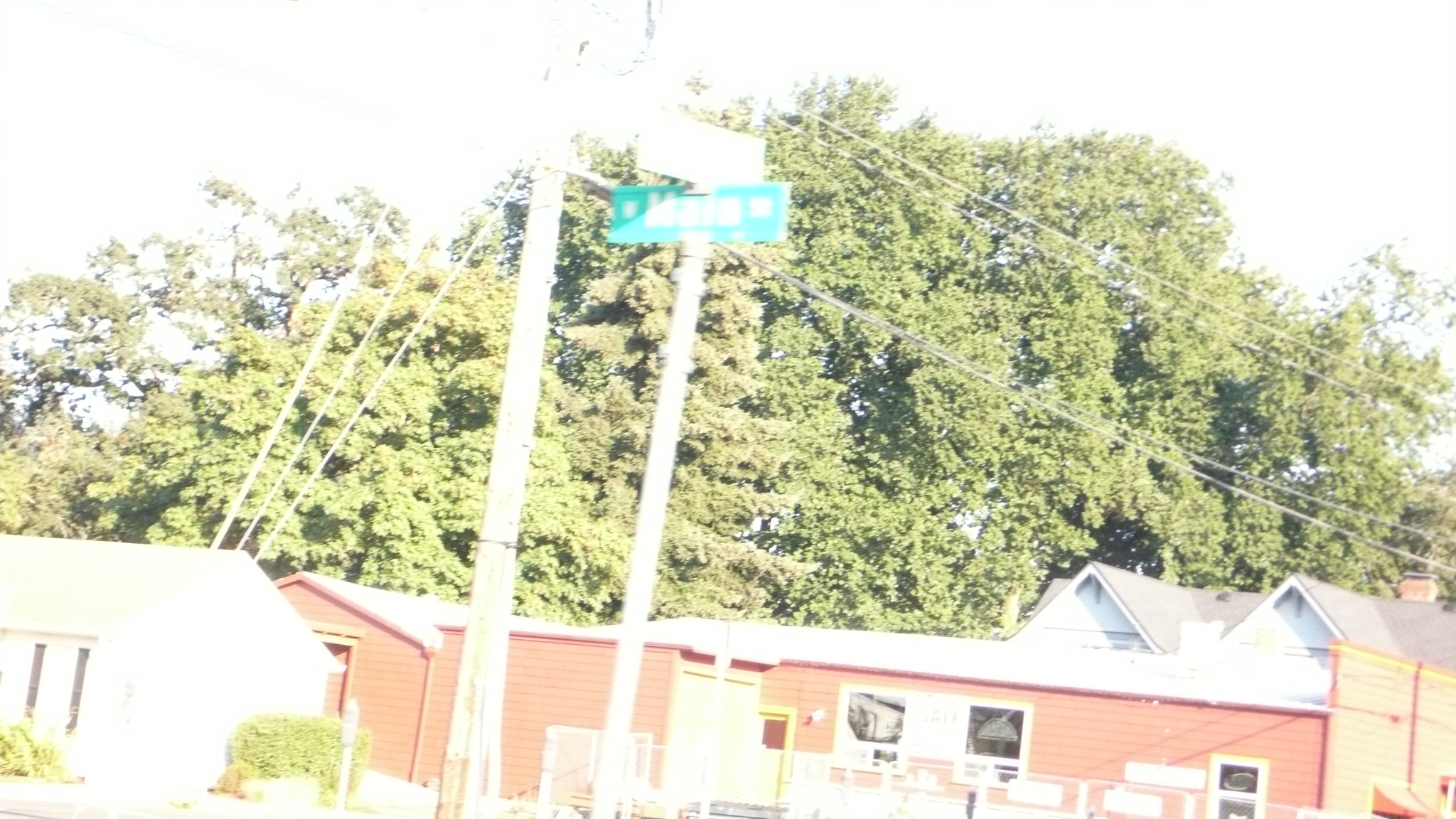This angled outdoor photograph captures a green rectangular street sign on a gray metal pole, with the word "Maine" displayed. The sunlight shines directly towards the sign, making the text hard to read. Behind the sign, a large wooden power pole stands, with numerous wires extending from the ground to the pole on the left and stretching across the scene on the right. 

In the left-hand side of the image, a small white building with an angled roof is visible. Central to the photo is a red house with a white roof and an attached garage. The background is filled with densely packed trees whose leaves and branches cover the entire upper part of the image, providing a lush, green backdrop. On the right side, a white house with a large wooden fence continues the residential setting.